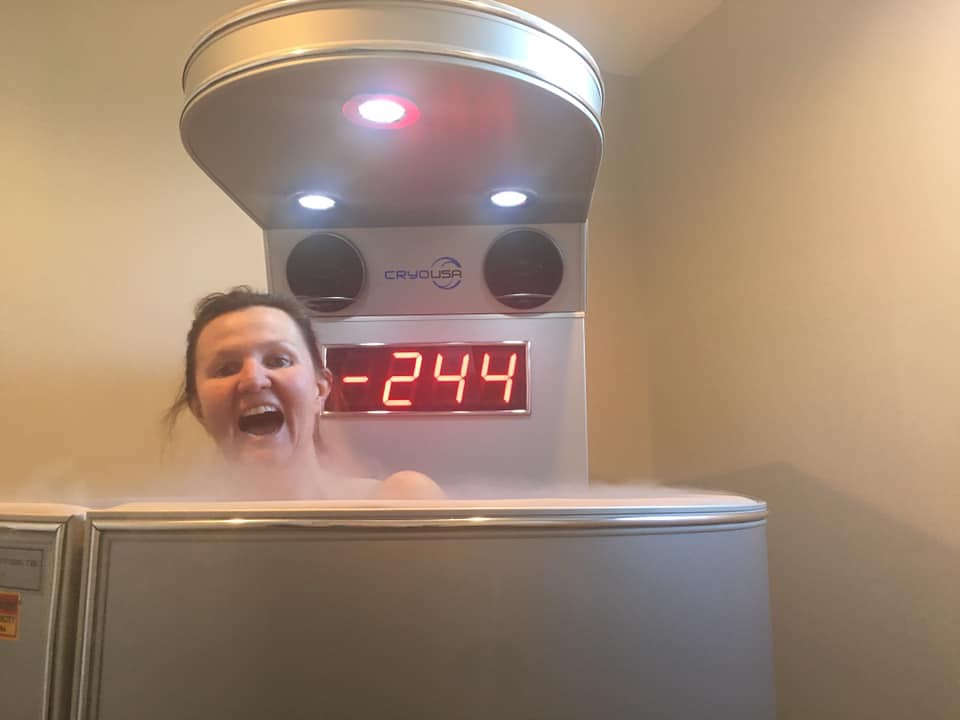In this detailed photograph, a woman with brown hair pulled back is immersed in a cryotherapy machine, branded with the text "Cryo USA" and a stylized globe graphic. The machine is designed like a large, round vat, located in a sharp corner where painted light white and gray walls meet. With her mouth wide open in a surprised expression, the woman’s bare shoulders are visible above the rim of the machine, from which multiple wisps of cold steam rise. An intricate structure extends from the back of the machine, featuring three lights on its overhang and a prominent LED display reading "-244."